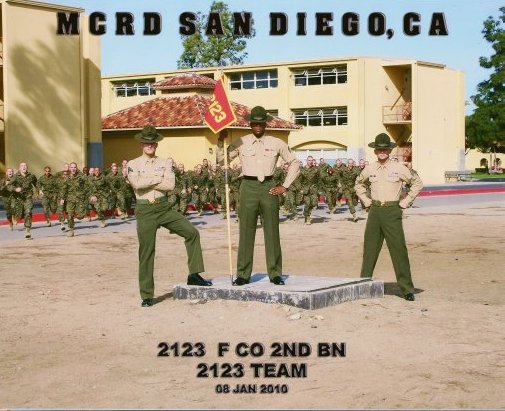In this detailed photograph, likely taken at a military training facility such as the Marine Corps Recruit Depot (MCRD) in San Diego, California, the sandy ground and yellow, multi-story barracks set the scene. The building, possibly housing or barracks, features numerous windows. At the top of the image, bold black text reads "MCRD, San Diego, CA." Below, three drill sergeants in green hats, tan button-down shirts, tan ties, and green pants stand prominently. The sergeant on the left has his arms crossed, the one in the middle holds a flag with "21-23" in his left hand, and the sergeant on the right stands with fists on his waist and elbows bent. Behind them, soldiers or recruits appear to be running in place with one foot in the air, mouths open as if chanting. Additional text centered at the bottom states "21-23 FCO 2nd BN," followed by "21-23 Team 08 Jan 2010," indicating the date and military unit.